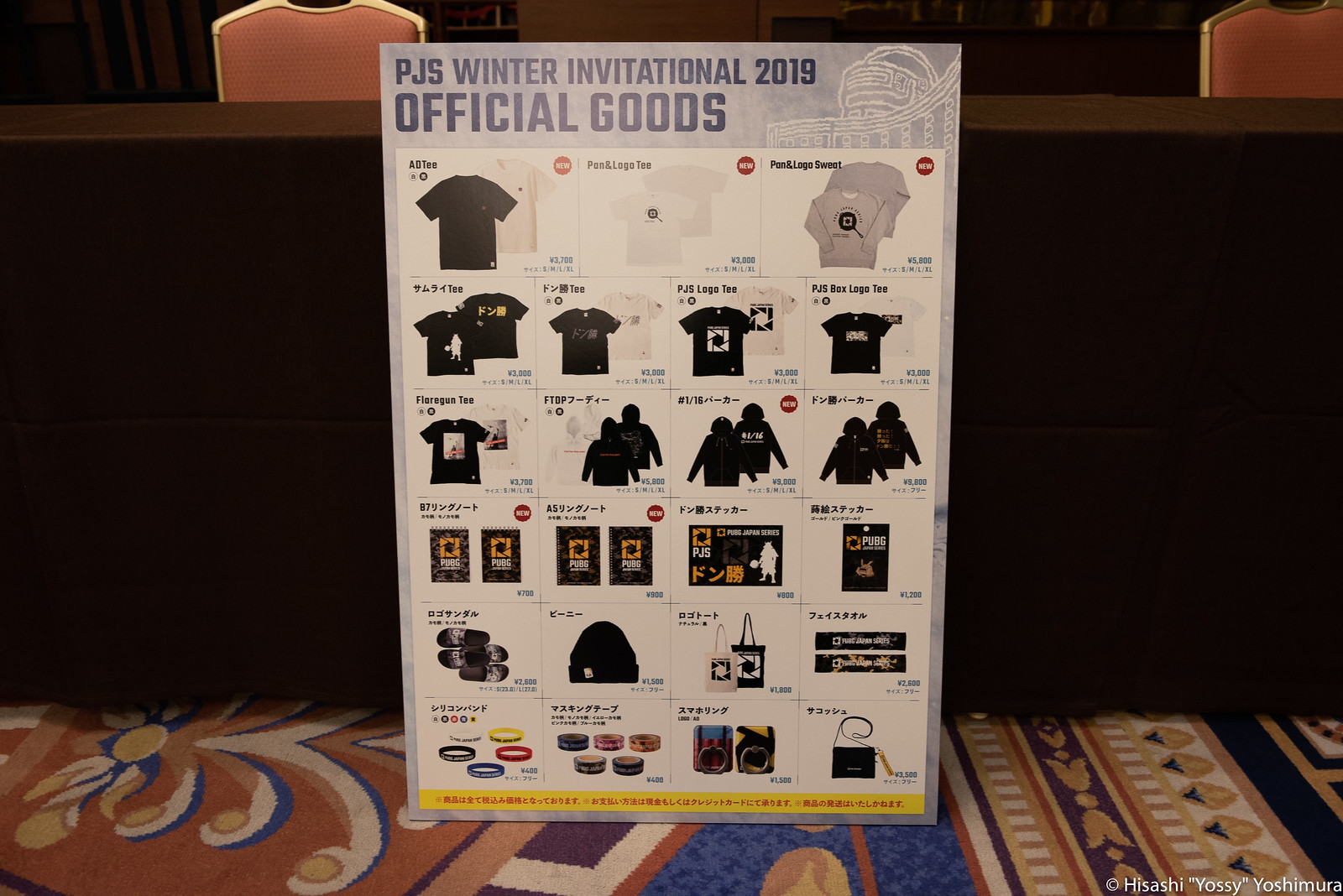This is a horizontal rectangular photograph capturing an indoor scene at a conference or similar event. The background is very dark and indistinct, with hints of hotel-like features such as multicolored carpet and off-red metallic-frame hotel chairs positioned behind a table draped in a long, dark cloth. At the forefront of the image is a sign with a gray background and a blue border across the top, showcasing the title "PJ5 Winter Invitational 2019 Official Goods." The sign displays an array of pictures representing various items available for purchase or as prizes, including t-shirts, hoodies, a purse, a handbag, shoes, and a beanie, all arranged in a four-by-three grid. The images come with descriptions and prices, some in English and some in what appears to be Korean or Japanese. The overall setting and signage suggest it is part of an official display for event merchandise.